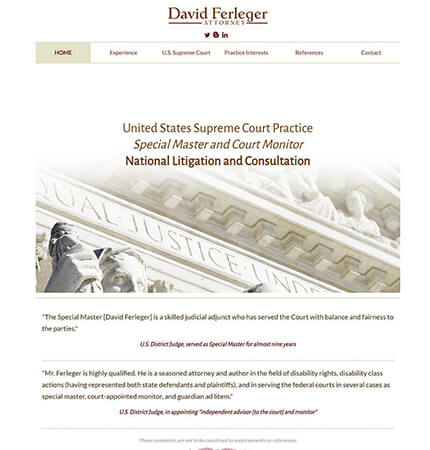**David Ferleger: Attorney at Law**

*Experience and Practice Overview*

This screenshot, possibly taken on a tablet given its dimensions, highlights the professional profile of David Ferleger, an esteemed attorney whose last name is spelled F-E-R-L-E-G-E-R. The interface includes several tabs such as "Home," "Experience," "U.S. Supreme Court Practice," "Interests," "References," and "Contact," with the "Home" tab currently selected. 

Beneath these tabs is a prominent grayscale image depicting the front of a court building embellished with the words "Equal Justice Under Law." Overlaid text reads: "United States Supreme Court Practice: Special Master and Court Monitor, National Litigation and Consultation."

*Testimonials*

Accompanying the visual elements are testimonials in small print that underscore Ferleger's distinguished career:

1. *“The special master, David Ferleger, is a skillful judicial adjunct who has served the court with balance and fairness to the parties,”* signed by a U.S. District Judge, noting that Ferleger has served as Special Master for almost nine years.

2. *“Mr. Ferleger is highly qualified. He is a seasoned attorney and author in the field of disability rights, disability class actions, having represented both state defendants and plaintiffs, and in serving the federal courts in several cases as Special Master, Court-appointed Monitor, and Guardian ad litem,”* cites another U.S. District Judge, who appointed him as an “independent advisor to the court and monitor.”

**Summary**

The composition of the screenshot and the accompanying testimonials reinforce David Ferleger’s extensive expertise in legal practice, with a notable emphasis on disability rights and his authoritative roles in the federal judiciary.